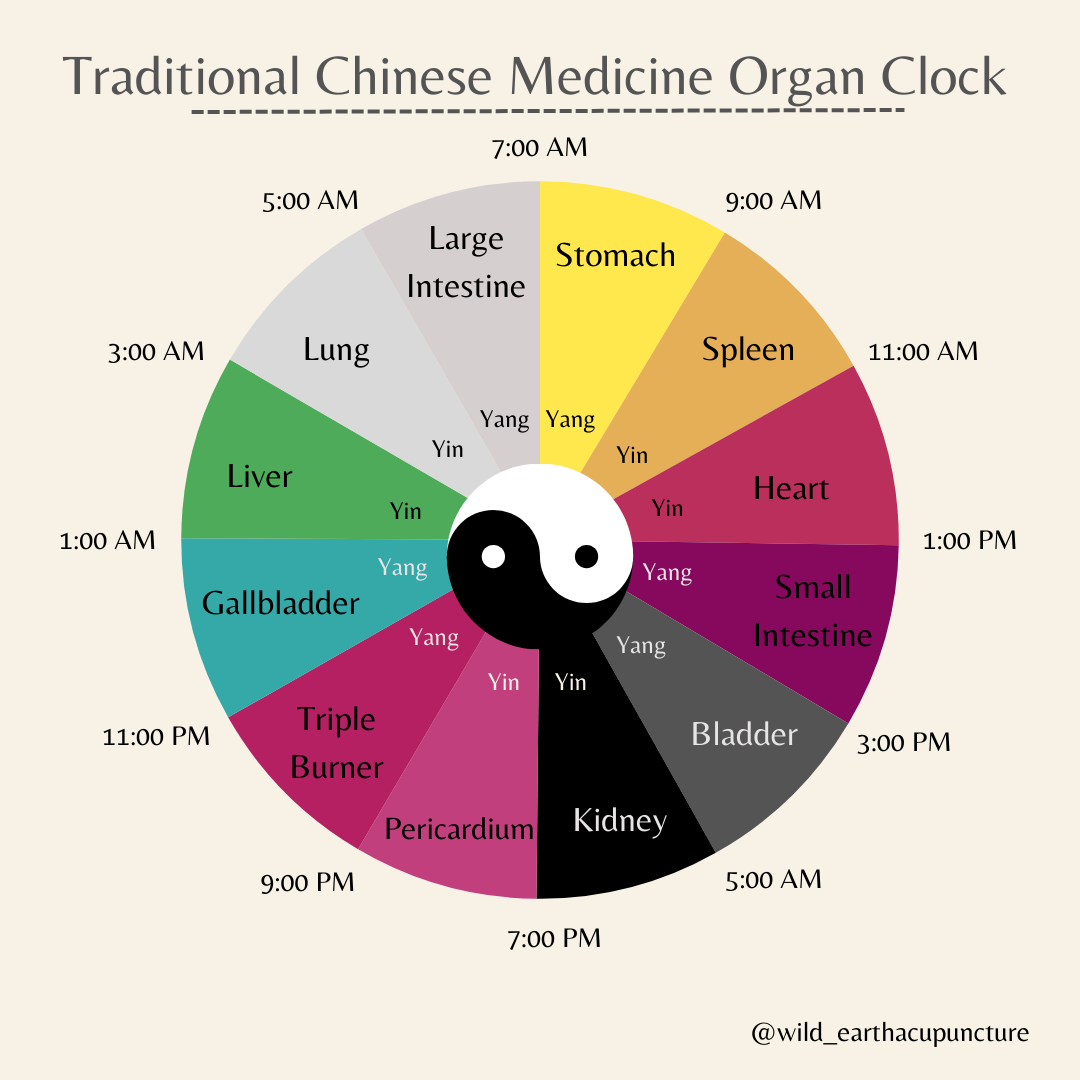This image features a detailed Traditional Chinese Medicine (TCM) organ clock on a white background, with "Traditional Chinese Medicine Organ Clock" written in black at the top and "at wild_earth acupuncture" at the bottom right. The clock is divided into 12 sections, each corresponding to a specific time frame, organ, and its yin or yang classification. 

- From 7 a.m. to 9 a.m., the yellow section represents the Stomach (Yang).
- From 9 a.m. to 11 a.m., the light brown section denotes the Spleen (Yin).
- From 11 a.m. to 1 p.m., the light red section is associated with the Heart (Yin).
- From 1 p.m. to 3 p.m., the purple section represents the Small Intestine (Yang).
- From 3 p.m. to 5 p.m., the gray section denotes the Bladder (Yang).
- From 5 p.m. to 7 p.m., the black section corresponds to the Kidney (Yin).
- From 7 p.m. to 9 p.m., the pink section represents the Pericardium (Yin).
- From 9 p.m. to 11 p.m., the cherry-red section is linked to the Triple Burner (Yang).
- From 11 p.m. to 1 a.m., the teal section signifies the Gall Bladder (Yang).
- From 1 a.m. to 3 a.m., the green section represents the Liver (Yin).
- From 3 a.m. to 5 a.m., the dark beige section denotes the Lung (Yin).
- From 5 a.m. to 7 a.m., the light gray section corresponds to the Large Intestine (Yang).

A central Yin-Yang symbol ties the diagram together, visually reinforcing the balance concept in TCM.